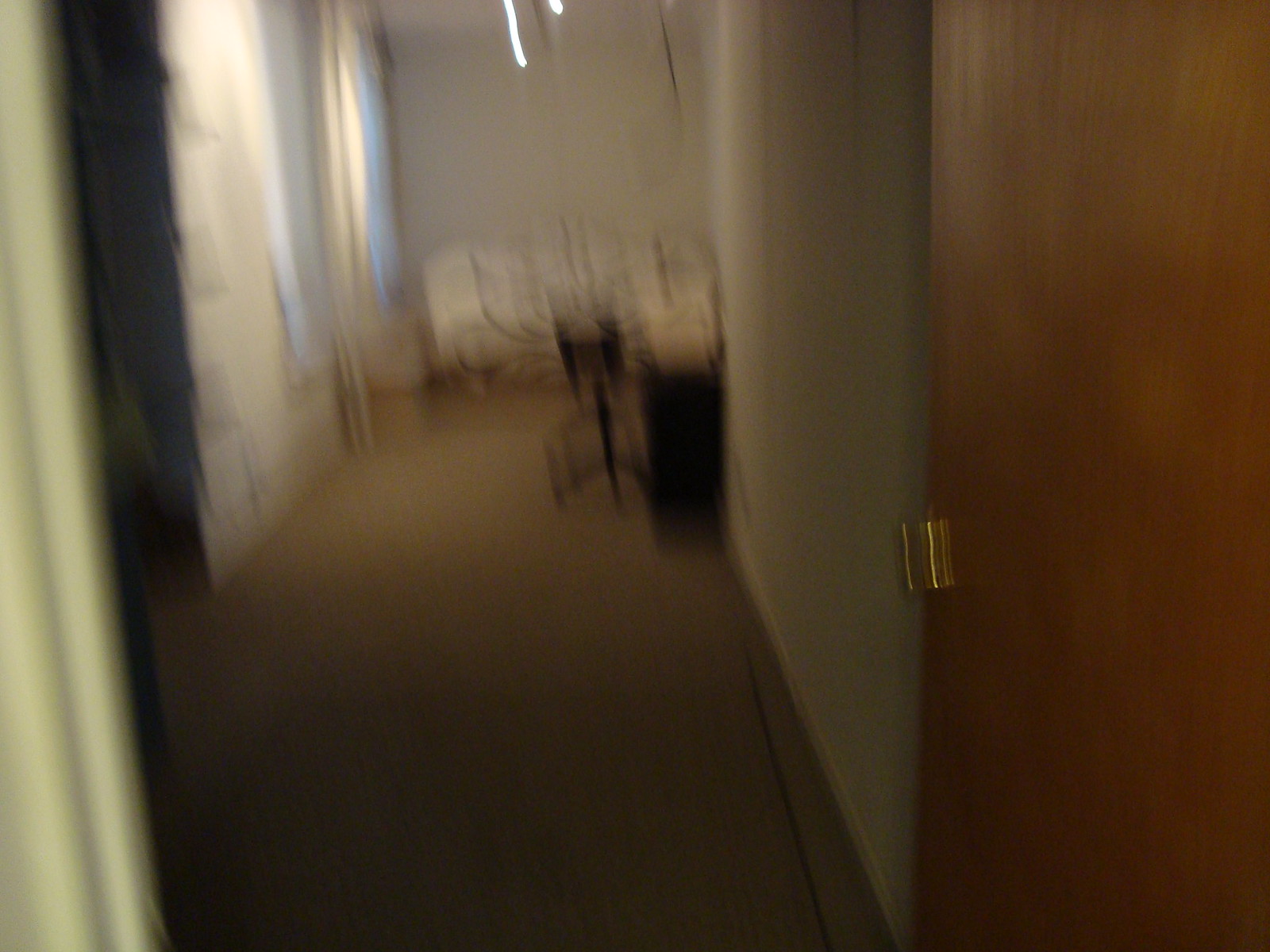The image, though very blurry, appears to depict either a hallway in an office or an entranceway into a room in an apartment or house. At the forefront of the image, directly ahead and down the hallway, there is a dark-colored object that possibly resembles a chair, though the blurriness makes identification difficult. This chair-like object has a leg structure that brings to mind an office chair, but it's not definitive. 

Adjacent to this potential chair, there's a very dark, short-standing cabinet, which seems to have some light-colored objects placed on top of it. The surrounding walls are light-colored, enhancing the visibility of certain features despite the blur. On the left side of the image, there are two windows allowing some blue-tinted light from outside to seep into the room, hinting at either early morning or dusk.

Further down the entranceway, past the chair and cabinet, there is a wooden door with a brown finish. This door is equipped with a gold handle, specifically a pole-style handle, which adds a hint of sophistication. The doorframe around it is of a light color, harmonizing with the hues of the surrounding walls.